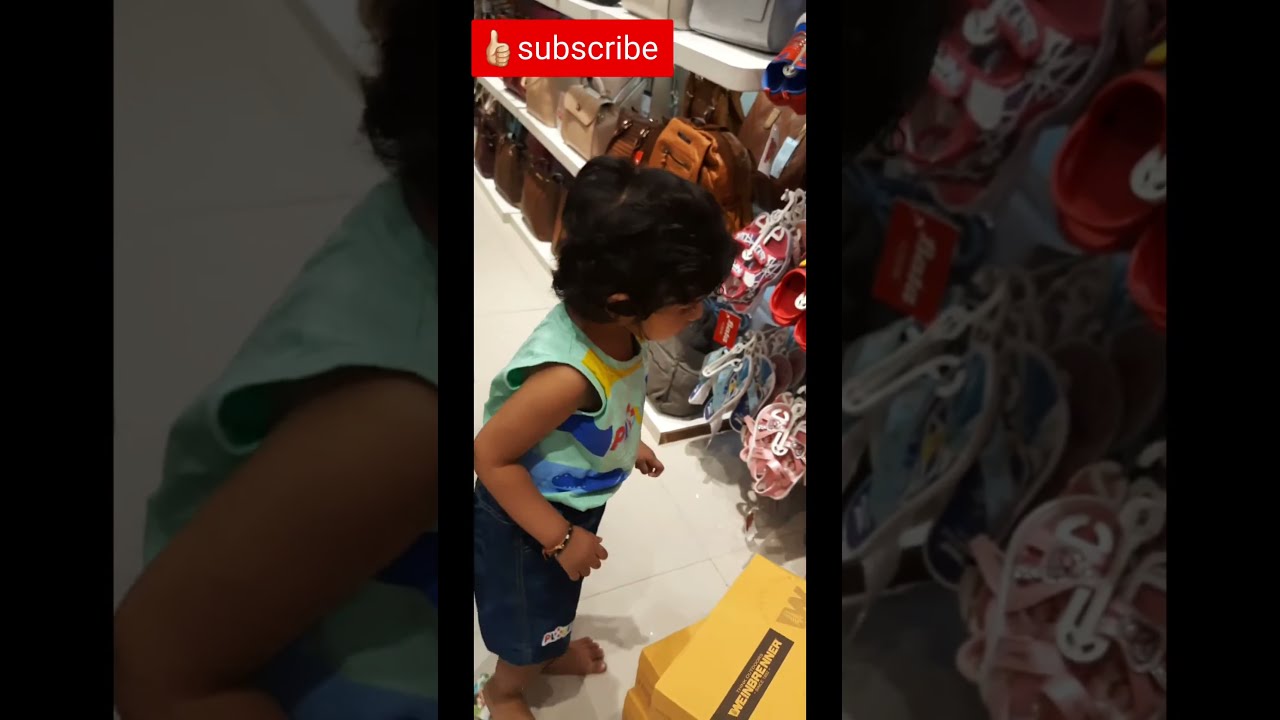The photograph captures the vibrant interior of a children's shoe store, where rows upon rows of bright-colored kids' shoes are meticulously displayed on white plastic hangers attached to the walls. The shoes vary widely in design, featuring styles reminiscent of Crocs, mini Converse, and other eye-catching patterns in hues of red, blue, yellow, orange, purple, and brown leather. The store's white floor provides a stark contrast to the explosion of colors surrounding it. In the foreground, two shoe boxes sit on the floor: one is yellow with black writing, and the other is tan in color.

Dominating the center-left of the image is a partial side profile of a child, whose small frame and attire are captured in detail. The child has black hair, tan skin, and is wearing a mint green tank top adorned with yellow and navy blue stripes. There is also mention of a curly-haired child wearing a similar tank top with light blue and deep blue stripes, indicating potential multiple perspectives of a single or different child within the image. The child’s facial features are mostly obscured, but a hint of curiosity can be inferred from their presence in the shoe-filled scene.

The image is noted to have sheer, black borders on both sides, which provide a zoomed-in, darkened close-up of the central scene, creating a distinctive framing effect. In the top portion of the photo, a 'thumbs up' sign and the word "Subscribe" are visible, adding an extra layer of context likely suggesting the image's use on social media or a video platform. Purses can also be seen arranged on a shelf to the upper left, adding another element to the retail setting. The overall composition combines to form a detailed and bustling snapshot of a child's shopping experience in a colorful shoe store.